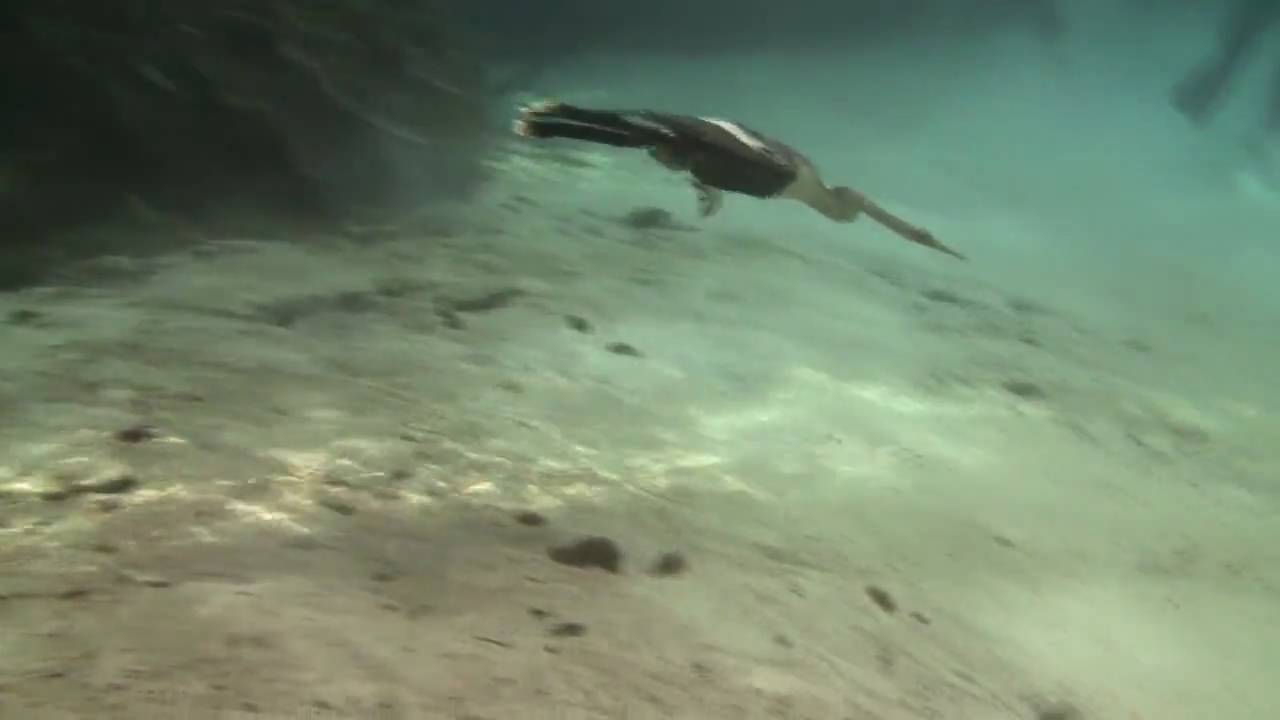This is a full-color, horizontally rectangular underwater photograph taken outdoors during the day, likely using a GoPro or phone camera. The image is quite blurry and poorly executed, with no discernible background aside from some sandy bottom and scattered rocks or vegetation. The sandy floor is light brown, dotted with several dark spots, which might be vegetation or sea urchins. In the upper left corner, there is an indistinct black area possibly representing a large rock structure or some other obscured object. The upper right corner shows part of a leg and a flipper, suggesting the presence of a diver. Central to the image is an elongated bird, underwater and likely swimming in a sleek, aerodynamic position as if diving for prey. The bird has a black body, wings, and head, with distinctive white markings on its back and neck, and a light-colored beak. The surrounding water has a blue-green hue, and there are scattered hints of black rocks or sea life on the sandy bottom.